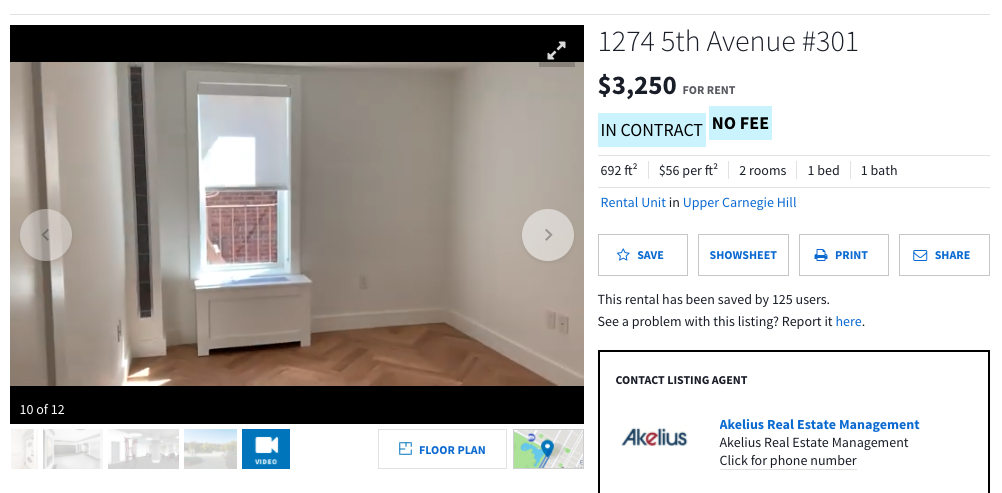This image is a detailed screenshot from a real estate listing, likely sourced from Zillow or a similar rental agency website. The image itself is framed by black bars at the top and bottom, with "10 of 12" indicated in white text at the bottom left corner. The center of the image features navigation arrows in gray within two small transparent circles, allowing users to click through additional photos.

The focal point of the image is a stark white room, notable for its pristine, minimalist aesthetic. A large window, framed and painted white, is positioned left of center, offering a glimpse of the outside. The floor of the room is covered in light tan wishbone-patterned parquet, adding a touch of elegance to the space.

On the right side of the image, the listing details are displayed against a white background in black and dark text. The property address is given as "1247 5th Avenue, Unit 302," with a listed rental price of $3,250 per month. Below this, in gray text, it states "4RAM" and "in contract," along with "no fees." The unit is described as having 629 square feet of space, translating to a cost of $56 per square foot, and includes two rooms: one bedroom and one bathroom. Additionally, in blue text, the listing specifies the unit is an "upper rental unit in Carnegie Hill."

Further down, user interaction options are provided: "Save," "Show Sheet," "Print," and "Share." It notes that this rental has been saved by 125 users. There is also a link for reporting issues with the listing, indicated in blue text. 

At the bottom right, there's a black square containing contact information for the listing agent. The text reads "Contact Listing Agent" in black, followed by "Lycos" and the company's name twice: "Lycos Real Estate Management," with a clickable link to reveal the phone number.